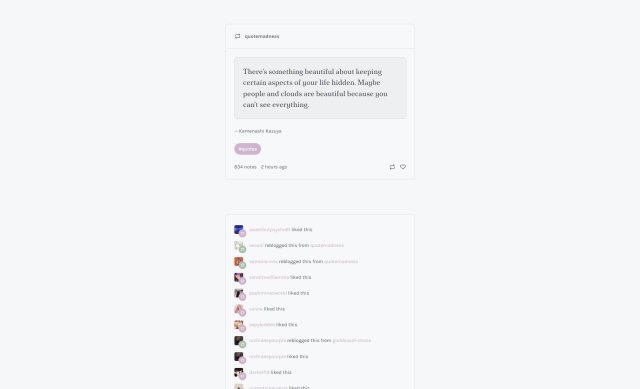This image appears to be a slightly unclear screenshot of a social media app on a phone. At the top, there's a header located in the top left corner beside a refresh icon. Below the header, a thin, gray horizontal line separates the header from the main content area. In the center of the image is a long rectangular box with a white background, containing a quote in a very small font that reads, "There’s something beautiful about keeping certain aspects of your life hidden. Maybe people or multiple people and something are beautiful because you can’t see everything." 

Following this text box, there seems to be some more text that is illegible, possibly providing additional context or commentary. Below this section, a medium-sized lilac-colored circle on the left side contains white text, although the exact words are unclear. The timestamp "two hours ago" indicates when the post was made. In the lower right-hand corner of the image, retweet and heart icons suggest options for interacting with the post, likely for sharing or liking it.